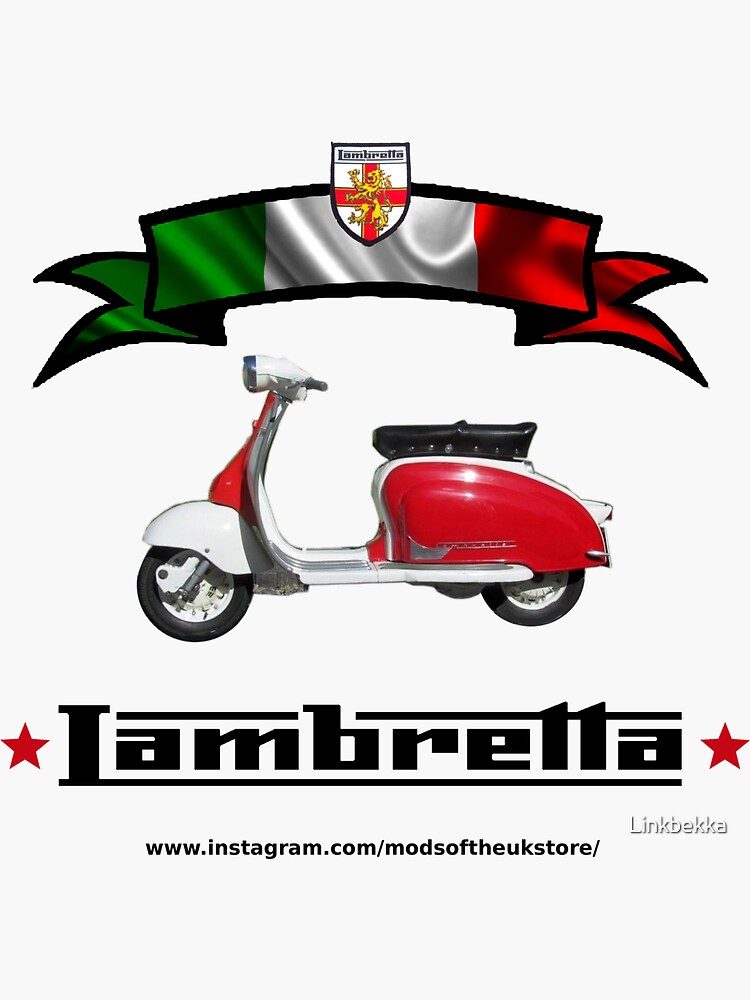The product image showcases a small red and white scooter, prominently featuring both colors across its body. The scooter's front neck and sides adjacent to the seat are red, while the top of the seat area is white. The black leather seat appears to be fastened with visible knobs or screws. The scooter is equipped with a headlamp at the front and rides on two black wheels. At the top of the image, a ribbon resembling the Italian flag—green on the left, white in the middle, and red on the right—serves as a backdrop to a prominent logo. The logo, shaped like a shield, features a red cross on a white background with a golden lion standing atop the cross. The text "LAMBRETTA" is inscribed above the lion within the shield. At the bottom of the image, the brand name "LAMBRETTA" is written in bold black letters flanked by red stars on both sides. Below this, an Instagram URL is provided: www.instagram.com/modsofukstore, with the word "link Becca" located at the bottom right-hand corner. The entire composition is set against a plain white background.